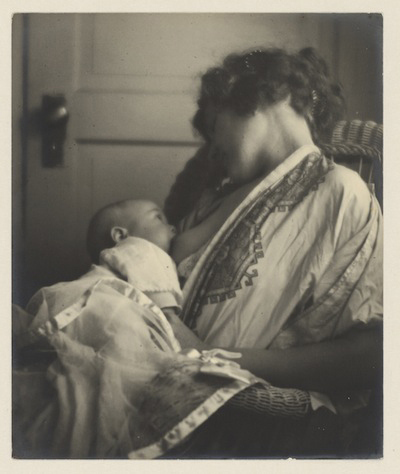The image is a beautifully vintage, sepia-toned photograph framed by a white border. It captures a tender moment of a mother breastfeeding her baby while reclining in a wicker chair. The scene is rendered with a moody, soft Gaussian blur, enhancing its timeless quality. The mother, dressed in a light-colored robe adorned with intricate patterning around the lapel, sits with a sheer blanket draped over her and the baby. Her head, adorned with dark, pinned-up hair, tilts away from the camera, and her eyes are closed as if she's asleep. Her right breast is exposed and the baby, dressed in light-colored clothing, is latched onto it, gazing up lovingly at the mother. This serene moment unfolds in front of a closed white door visible in the background, contributing to the photograph's overall intimate and nostalgic feel.